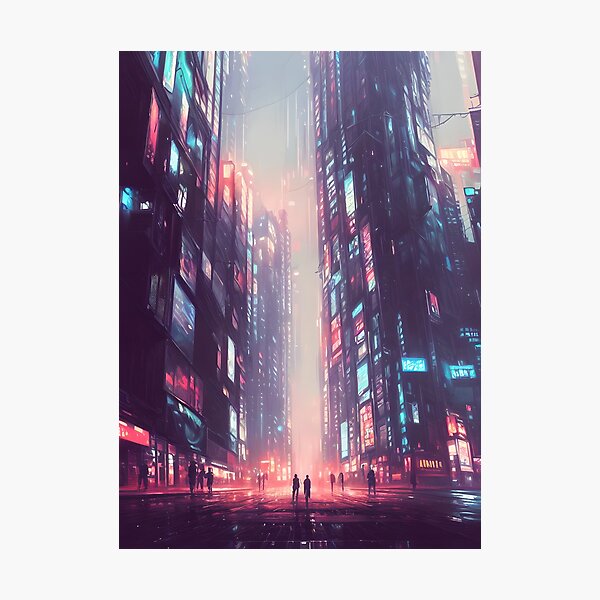The image is a vibrant, highly stylized representation of a sci-fi cityscape, featured as a product poster. It is a small, rectangular picture with the sides being twice as long as the top and bottom, floating against a flat, white background to focus attention solely on the artwork. The scene depicts a night-time urban street, with two small figures standing in the middle of the road and others ambiguously placed on the sidewalks. Tall, almost surrealistic buildings lined with an array of LED billboards, displaying generic patterns of blues, reds, and whites, tower both sides of the street. On the right, a partially visible skyscraper adorned with neon signs and lit windows stretches beyond the frame. The wet street, implying recent rainfall, reflects an orange glow around the figures, enhancing the sense that the area is illuminated by numerous video displays. The overall aesthetic evokes a dreamlike, futuristic environment with an emphasis on vibrant, unreal colors and a hazy, atmospheric quality.